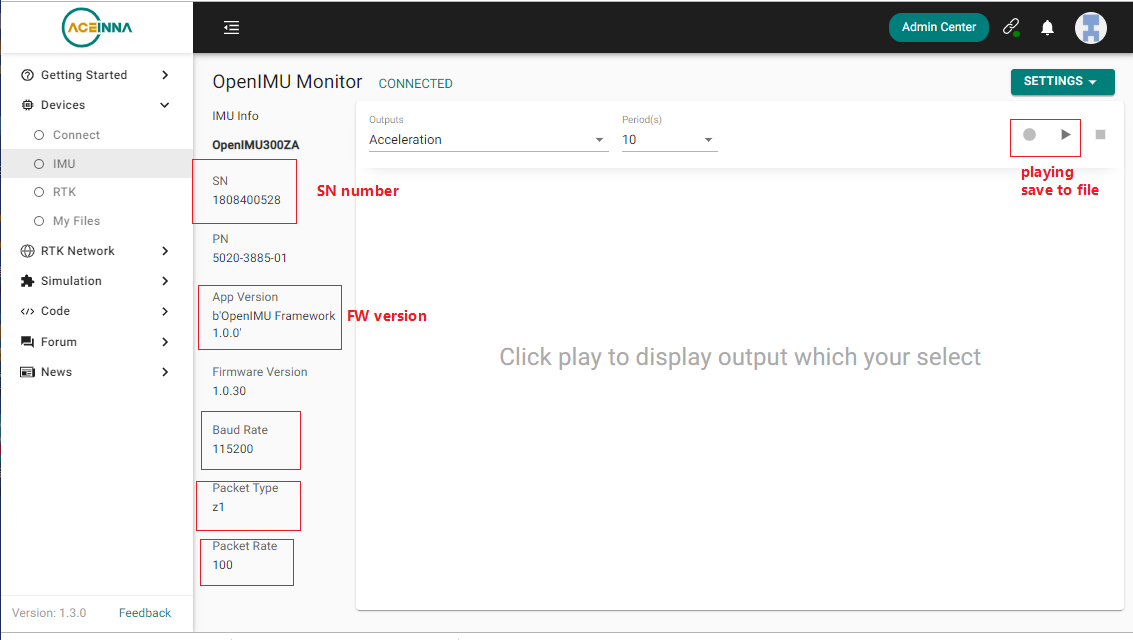Here is the cleaned-up and detailed descriptive caption for the desktop application screenshot:

---

The screenshot displays an interface of a desktop application named "ACEINA." Positioned at the top left, the application name "ACEINA" appears in a combination of colored letters: "ACE" is in vibrant orange, while "INNA" is in a greenish hue. The prefix "ACE" is partially enclosed within an orange circle reminiscent of a Pac-Man figure.

To the right of the application name is a series of icons and buttons. First, there is an "Admin Center" button, styled as a blue-green pill-shaped icon. Following this, there is a chain-like symbol, likely indicating an attachment or link feature. Next to the chain icon is a notification bell, and adjacent to that, a placeholder for the user's profile image, currently showing a generic image in the absence of a user-uploaded picture. Directly below the notification bell and the profile placeholder is a settings drop-down menu button.

Further down the interface, a red rectangle with a white background contains play and record buttons. Below this, the text reads "Playing, save the file," with a square stop button located to the immediate right of this section.

Towards the middle left of the interface, there is an option labeled "Open IMU Monitor," followed by "IMU Info." The subsequent text reads "Open IMU 300-ZA," with additional details listed below, including serial number (SN), part number (PN), app version, firmware version, baud rate, packet type, and packet rate.

In the center of the interface is an instructional message on a predominantly white background, stating: "Click play to display the output you select." At the bottom left corner, the software version number "1.3.0" is displayed. Finally, to the right of the version number is a greenish hyperlink labeled "Feedback."

---

This detailed description encapsulates the visual layout and functionalities of the desktop application interface as depicted in the screenshot.